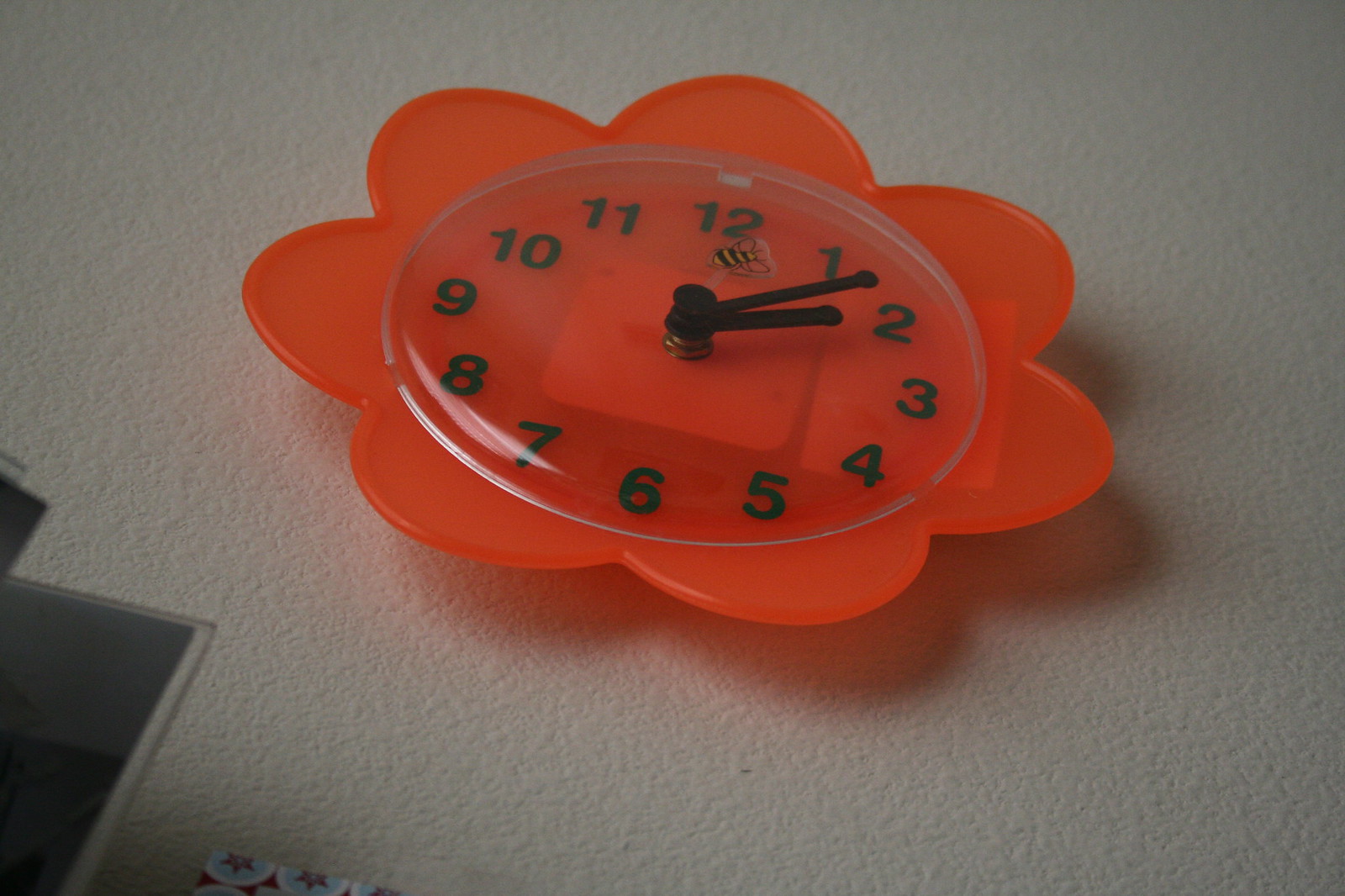A charming, child-friendly clock is mounted on a plain white wall, casting soft shadows with its whimsical frame. The clock's design is simple yet playful, with an orange flower-shaped frame that appears to be made of plastic. The timepiece is shielded by a transparent cover, likely made of glass or plastic. At the center of the clock, a cheerful illustration of a buzzing bee adds a delightful touch. The clock features Arabic numerals and its short black hour and minute hands are both positioned at the two o’clock mark. The overall aesthetic and design suggest this clock is perfectly suited for a child’s room or nursery.